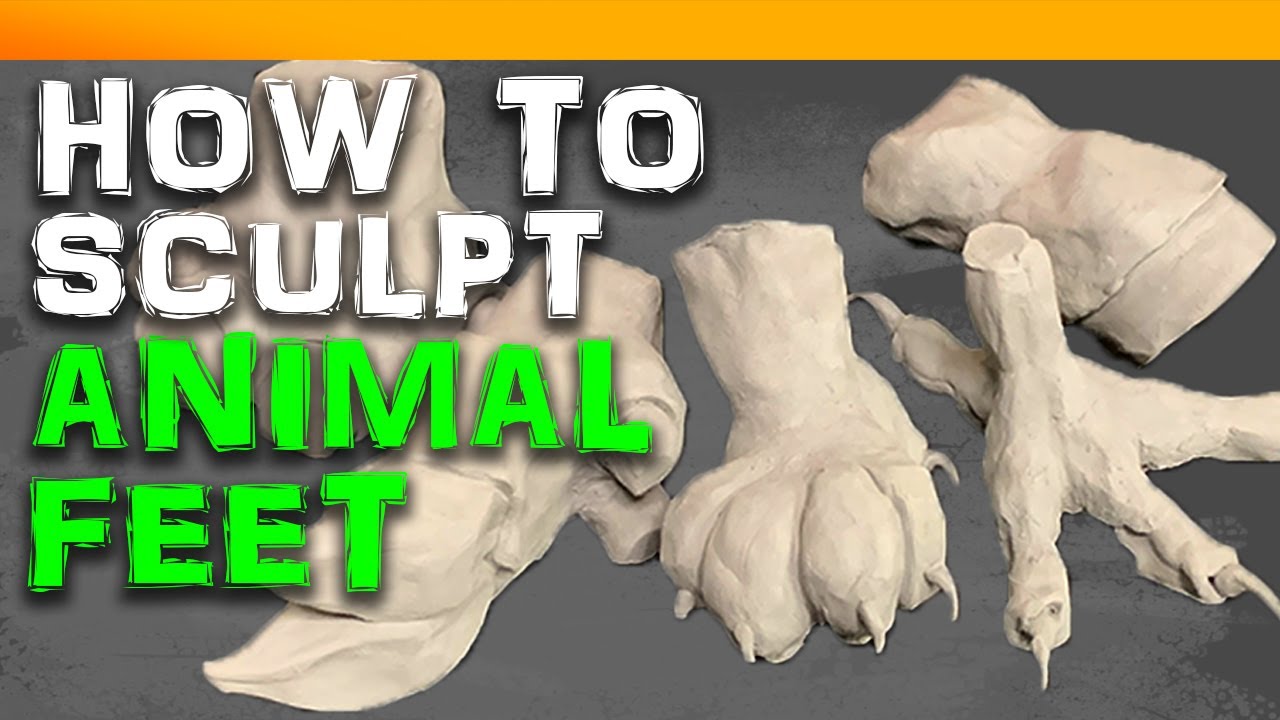The image features a detailed display of various animal feet sculpted from beige clay, set against a charcoal gray background. These lifelike clay models showcase intricate details, including what appear to be a bird's foot with spiky toes and long claws, and a dog's paw, complete with short fur and sculpted nails. The upper part of the image is bordered by a tangerine-colored strip. Superimposed over the feet are the words "How to Sculpt Animal Feet" in block letters, with "How to Sculpt" in white and "Animal Feet" in chartreuse green. Some portions of additional animal feet and parts of the text are obscured, making precise identification of all the sculptures challenging. This image likely serves as a guide or instructional piece for sculpting realistic animal feet.